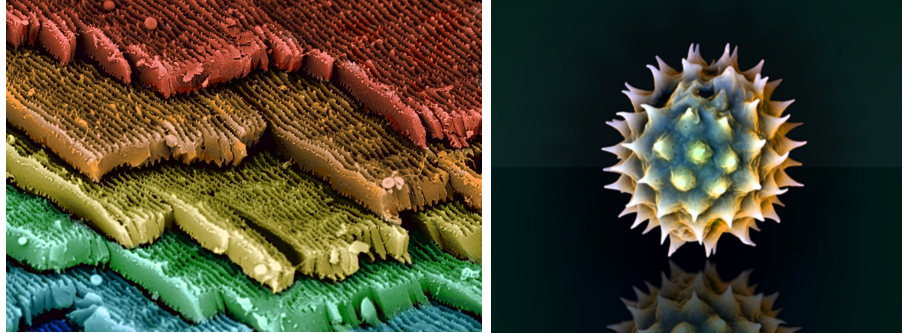The composite image features two highly magnified views, each presenting unique details and vibrant colors. On the left, layers of material reminiscent of fibrous structures or possibly wax, are arranged like a staircase to reveal multiple tiers. These layers are distinctly colored in a sequence from top to bottom: red, orange, yellow, green, and blue. The texture varies from smooth to rough across the layers, suggesting the image may have been artificially colored for better differentiation under the microscope.

The right-hand image showcases a spherical object resembling a virus or similar microorganism. This object is adorned with numerous spikes protruding from its surface, creating a thorny appearance. It is predominantly colored in shades of blue and yellow, with accents of gray and purple, set against a stark black background. The artificial coloring enhances the contrast, making the intricate details and texture of the spiked sphere more visible.